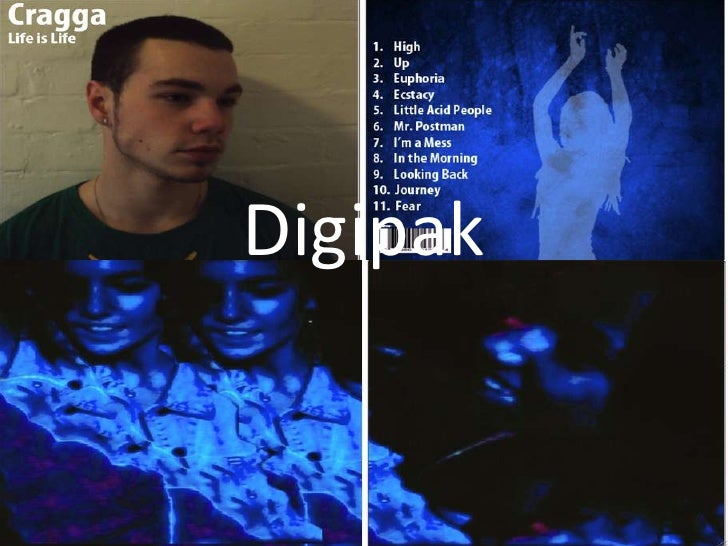The image is a detailed collage of an album cover and its components, presumably for the album "Life is Life" by the artist Craiga. The top left segment features the main album cover, displaying a close-up of a middle-aged man with short black hair and a slight shadow from stubble. He is looking to the right, dressed in a green shirt and a necklace, with a silver earring in his ear. White text near the top left corner reads, "Craiga, Life is Life," likely indicating the artist's name and album title. 

The top right segment of the collage appears to be the back cover, showcasing a blue-tinted image of a woman with long hair, her hands raised in a dancing pose. This section also contains the track listing for the album, numbered from 1 to 11 with titles: High, Up, Euphoria, Ecstasy, Little Acid People, Mr. Postman, I'm a Mess, In the Morning, Looking Back, Journey, and Fear. A barcode is placed beneath these titles, partially obscured by the white text "Digipak" printed in the center.

The bottom left portion of the collage reveals the inside of the album, featuring a blue-hued image of two women's faces above an indistinct object. Meanwhile, the bottom right segment displays a heavily abstract and distorted blue image where a female face is barely discernible. The entirety of the collage is dominated by a blue tint, giving it a cohesive aesthetic style.